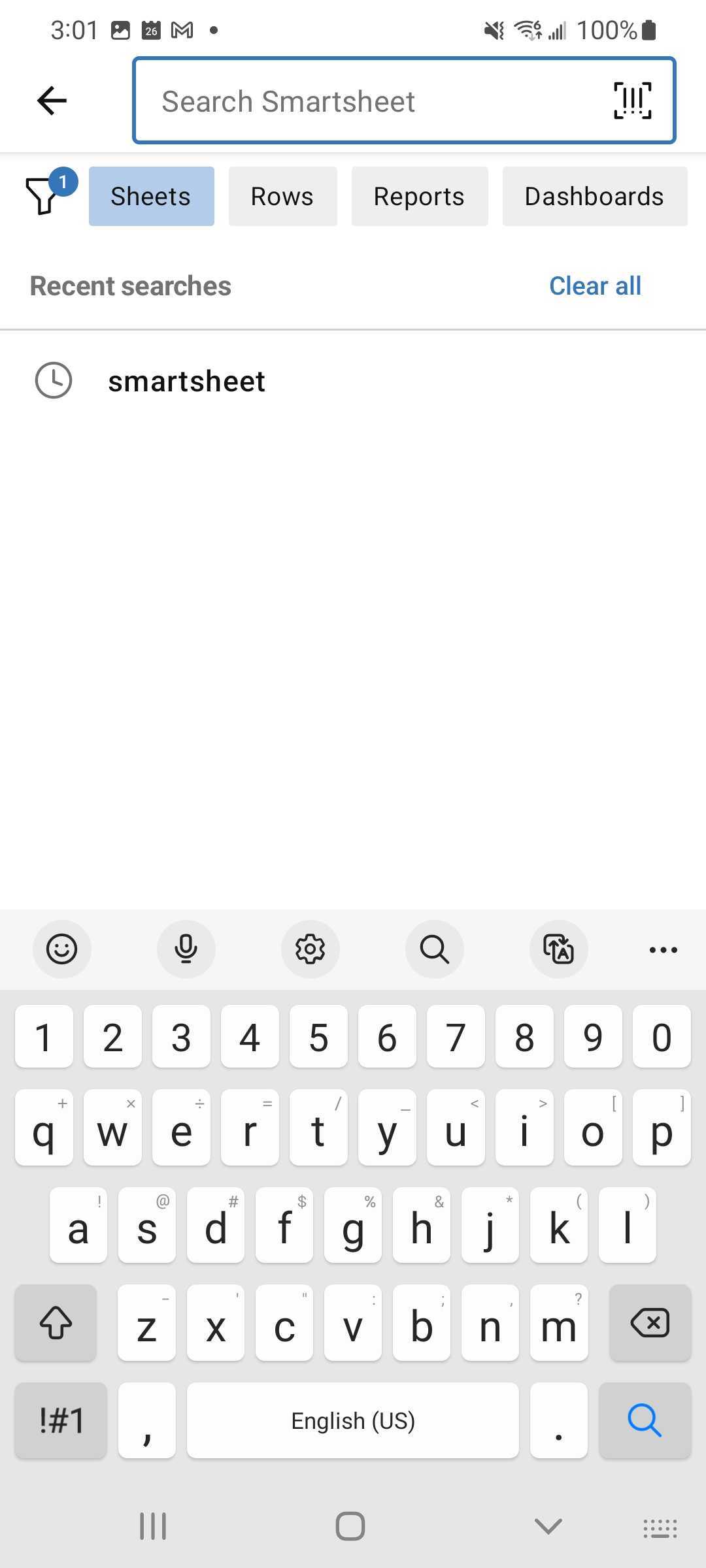The image showcases a digital device screen with several interface elements arranged in a structured manner. In the top left corner, there are multiple icons including a clock displaying "3:01", a picture icon, a calendar icon, and a mail icon. Moving to the top right, a series of additional icons are visible: a mute icon, a Wi-Fi icon, a cellular signal icon, and a battery icon showing "100%". Below these icons lies a search bar that contains the text "Search Smartsheet". Adjacent to the search bar on the right is a barcode icon, and on the left, a back-arrow icon.

Directly beneath the search bar, a horizontal menu displays various options: a filter icon on the left followed by the labels "Sheets", "Rows", "Reports", and "Dashboards". Below this menu, on the left side of the screen, there is a section labeled "Recent Searches", while on the right side, a "Clear All" option is present. At the bottom of the screen, the word "Smartsheet" is prominently displayed, suggesting that the interface belongs to the Smartsheet application.